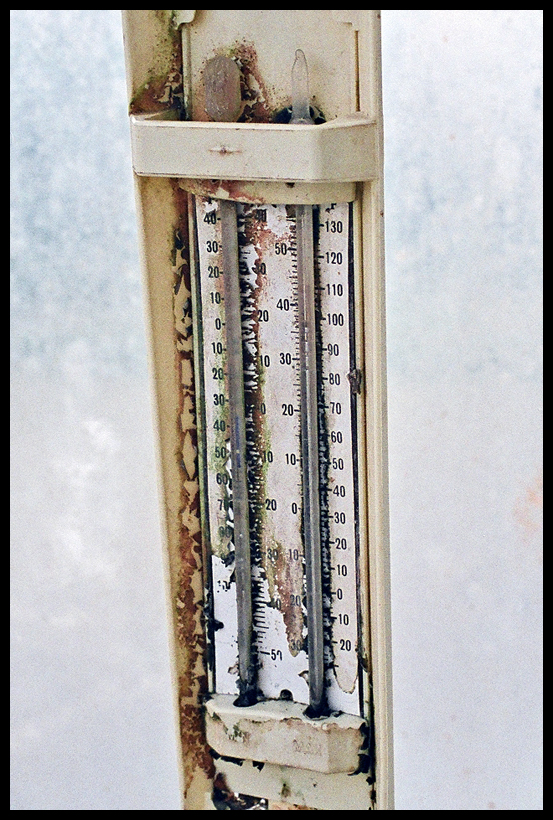This photograph prominently features two aged thermometers, each set against a backdrop of a bluish-white band reminiscent of a sky with clouds. Positioned centrally, the primary thermometer showcases a weathered appearance with an off-white, rusted metal base. Rust streaks down the left side of this thermometer, transforming areas of the metal into a rusty brown hue. At its apex, a horizontal metal band and an exposed thermometer flask are visible.

The midpoint of this primary thermometer is marked by a white label displaying temperature measurements, reading from -20 to 130 degrees Fahrenheit. Just to the left, a second thermometer is positioned, albeit in a more deteriorated state. Its base is similarly aged, and its numbered measurements, beginning faintly at 51, appear significantly faded and partially worn away. The combination of these elements creates a nostalgic depiction of vintage instrumentation against a serene backdrop.